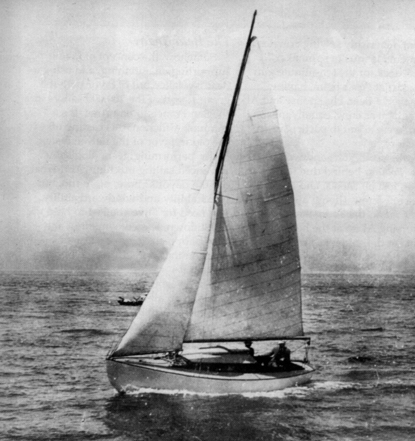The image is an older, black and white photo with a grainy quality. It depicts a small sailboat on the ocean, framed by a cloudy sky. The sail is unfurled, and if you look closely, you can make out a person at the bottom, back end of the boat, shadowed by the sail. The water surrounding the boat has a white appearance. In the background, another small boat without visible sails can be seen.